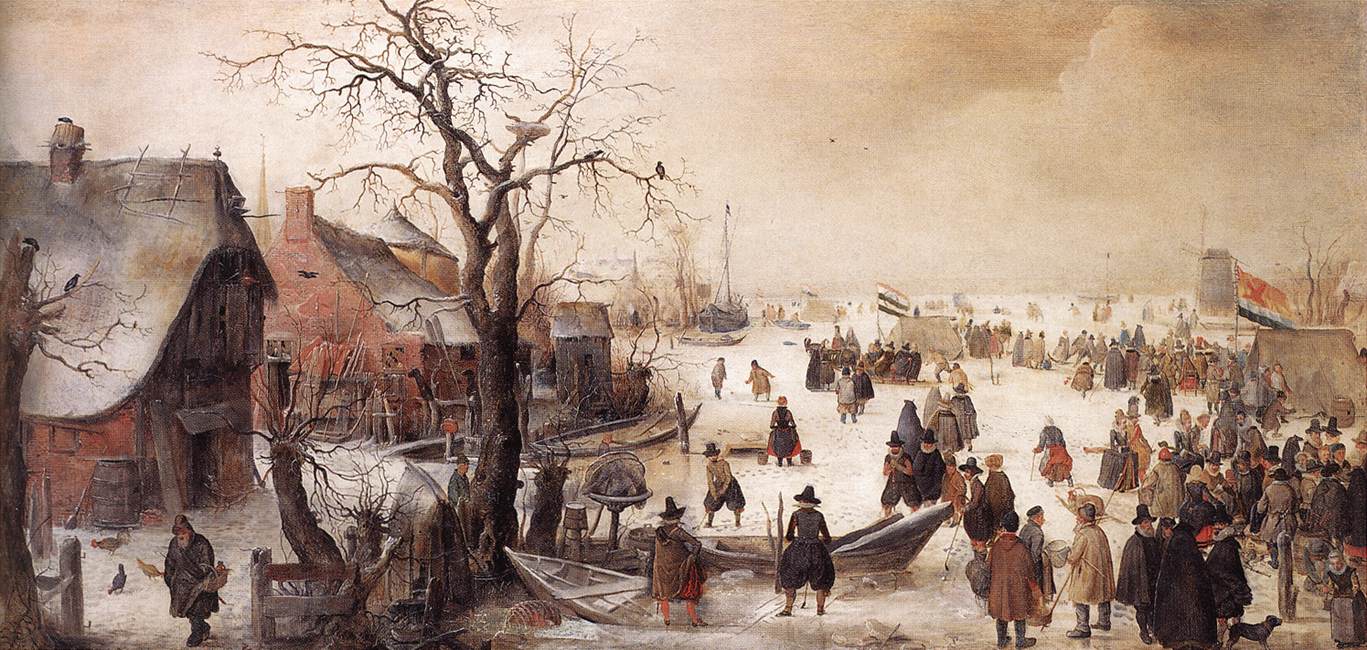This color landscape oil painting titled "Winter Scene on a Canal" by Hendrik Averkamp vividly depicts a small, bustling Dutch village during the wintertime in the 1600s or 1700s. The scene captures a snow-covered landscape with several rudimentary wooden and brick houses with sloping thatched roofs on the left. Prominently, a large, barren oak tree stands about a third of the way from the left, adding to the wintry atmosphere. In the foreground, traditional Dutch attire, including pantaloons and tall hats with buckles, adorns the villagers, who congregate and converse. Children play on the partially frozen canal while adults navigate around canoes.

The background of the painting features several windmills and ice-bound boats, emphasizing the harsh winter condition. A group of people, including those waving a Dutch flag, can be seen in the center, adding a multinational element with other flags possibly representing the Irish among them. The sky above is ominous with shades of gray and beige, suggesting an impending snowfall. This detailed scene is filled with nearly 100 figures, mostly men, illustrating life in a Dutch town during a cold, winter day in the historical style that Averkamp is known for.